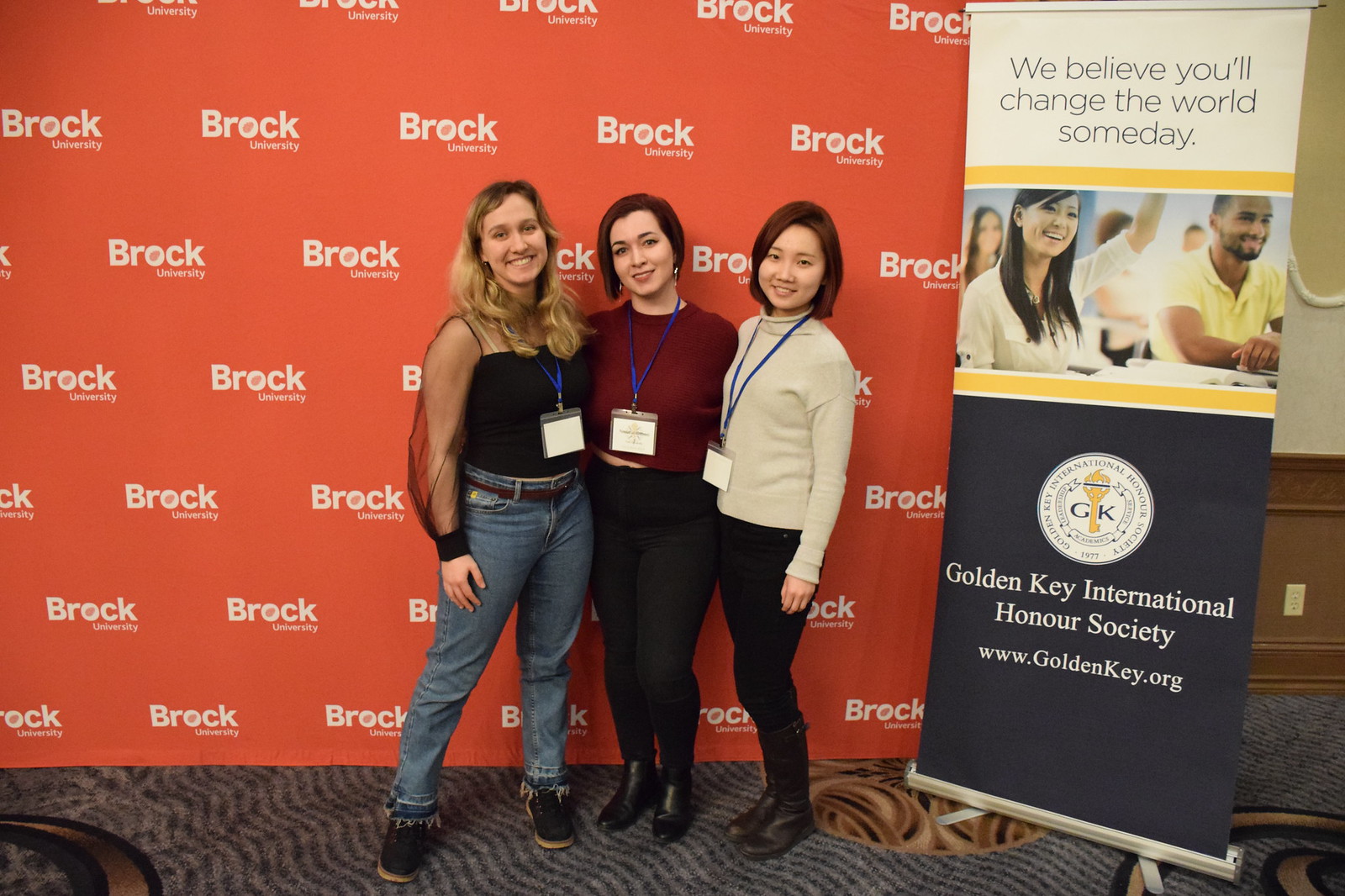In this vibrant color photograph, three young women are standing closely together on a gray rug, facing the camera and smiling. Each woman is wearing a lanyard around her neck, conveying a sense of camaraderie and uniformity. The woman on the left has blonde hair and is clad in a sheer black top with long sleeves, blue jeans, and black shoes. Standing next to her, the woman in the middle has short black hair and is wearing a burgundy t-shirt paired with black pants and shoes. On the right, the third woman also with short black hair is dressed in a cream sweater, black pants, and black shoes. 

The background features a prominent orange banner repeatedly emblazoned with the white "BROCK UNIVERSITY" logo, indicating their affiliation or location. To the right of the trio is a detailed stand-alone poster. This poster bears the inspirational message, "We believe you'll change the world someday," and includes an image of two smiling students. Below this, the poster displays the circular logo of the Golden Key International Honour Society, accompanied by its name in white letters and a website link. The image exemplifies photographic realism, capturing the warmth and optimism of the moment.